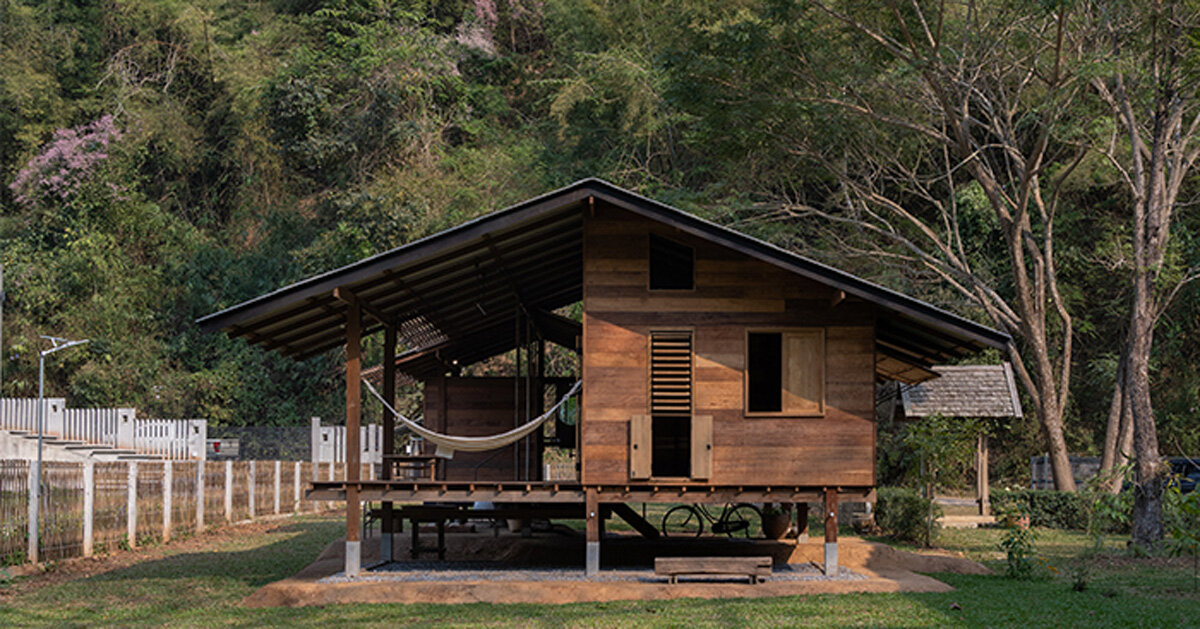This landscape photograph captures a charming wooden cabin nestled in the midst of a lush green forest. The cabin, elevated on metal stilts above a layer of gray gravel, blends rustic charm with modern touches. The structure features a metal roof that extends over both an enclosed section on the right and a spacious deck on the left. The deck is adorned with a hammock hanging between a pole and the cabin, making it an ideal spot for relaxation. White mesh or metal fence posts line the left side of the image, adding a touch of quaintness. Surrounding the cabin is vibrant green grass, and the backdrop is filled with a dense canopy of tall trees with leafy branches. A small lean-to structure supported by four posts is situated on the right side of the cabin, adding to the cozy atmosphere. Notably, a bicycle peeks out from underneath the cabin, hinting at outdoor adventures. Additional details include a window and a small door on the right side of the cabin, further enhancing its inviting appearance.